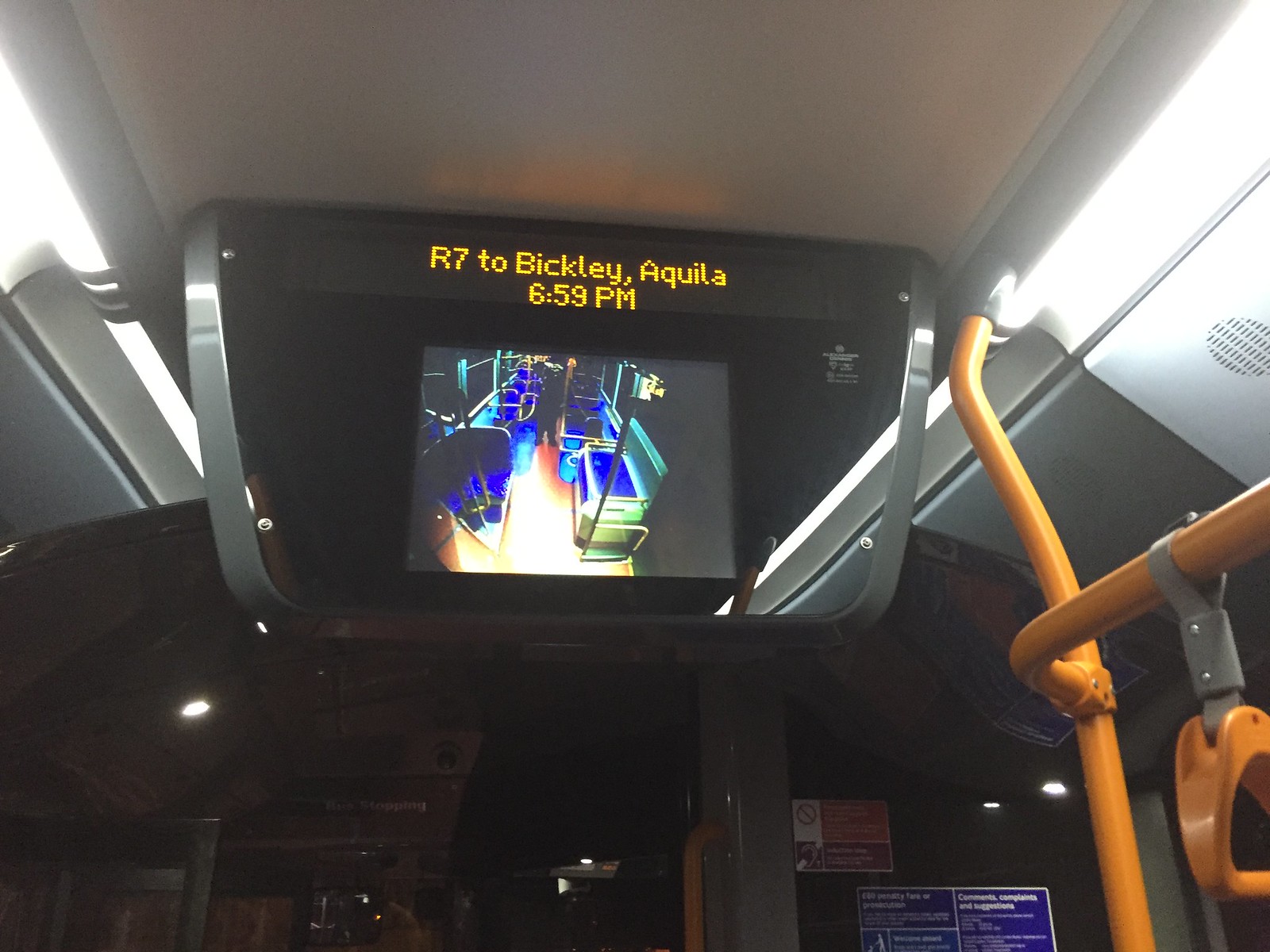The image depicts the interior of a public transportation vehicle, likely a subway car or bus, taken at night. A prominent focal point in the photo is a ceiling-mounted screen displaying a live feed from a security camera, showing a corridor with blue empty seats and the shadowy figure of a person. The time indicated on the screen is 6:59 p.m., with the route marked as "R7 to Bickley Aquila" in bright orange text on a black background. 

The vehicle features orange and yellow horizontal bars interspersed with gray straps for passengers to hold onto. The ceiling and upper walls are white with silver accents, while the floor and some bars contrast in orange. A non-smoking symbol is visible on one of the walls, emphasizing a no-smoking policy with a red slashing line over a white background. The overall lighting is dim, casting a shadowy and somewhat unfocused ambiance throughout the vehicle.